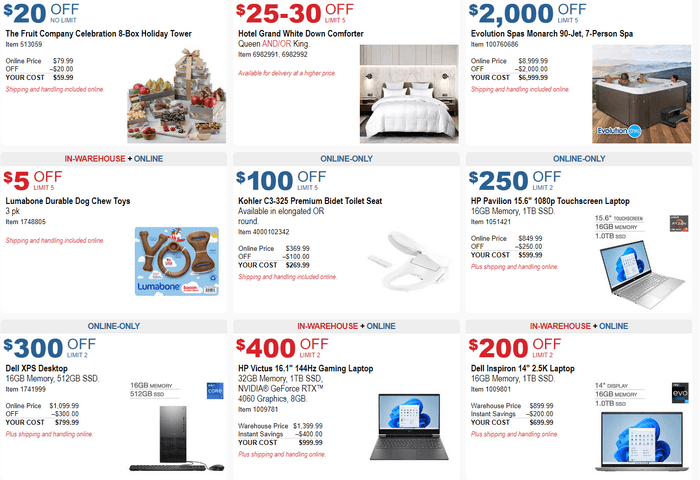The image depicts an array of colorful advertisements displayed on a wall, set in a grid pattern with three rows and three columns, totaling nine individual ads. These advertisements seem to offer various products and discounts, typically found in a warehouse or online catalog. 

In the top-left corner is an ad promoting a fruit company's "8 Box Holiday Tower." Originally priced at $79.99, the promotion offers a $20 discount, reducing the final price to $59.99, with shopping and handling included.

Adjacent to this, another ad showcases a hotel-grade "Grand White Down Comforter." The discount here ranges from $25 to $30, with a purchase limit of 6 units. The comforter is available in both Queen and King sizes, though prices may vary based on delivery options.

On the bottom row, an ad displays a luxurious "Evolution Spa" with 90 jets, accommodating up to 7 people. The online price is listed as $8,999.99, but a substantial $2,000 discount brings the cost down to $6,999.99, subject to a limit of 5 purchases.

Another notable ad offers $5 off on a three-pack of "Lumbar Bone Durable Dog Chew Toys," again with shopping and handling included in the final price, and a purchase limit of 5.

Finally, there's an ad for a "Kohler 3 C3" with a staggering $100 discount, also limited to 5 units.

Overall, the grid of ads highlights a diverse range of products, from luxurious comfort items to pet supplies, all accompanied by significant discounts. There's no visible website information provided, implying the offers are for a certain location or exclusive membership platform.